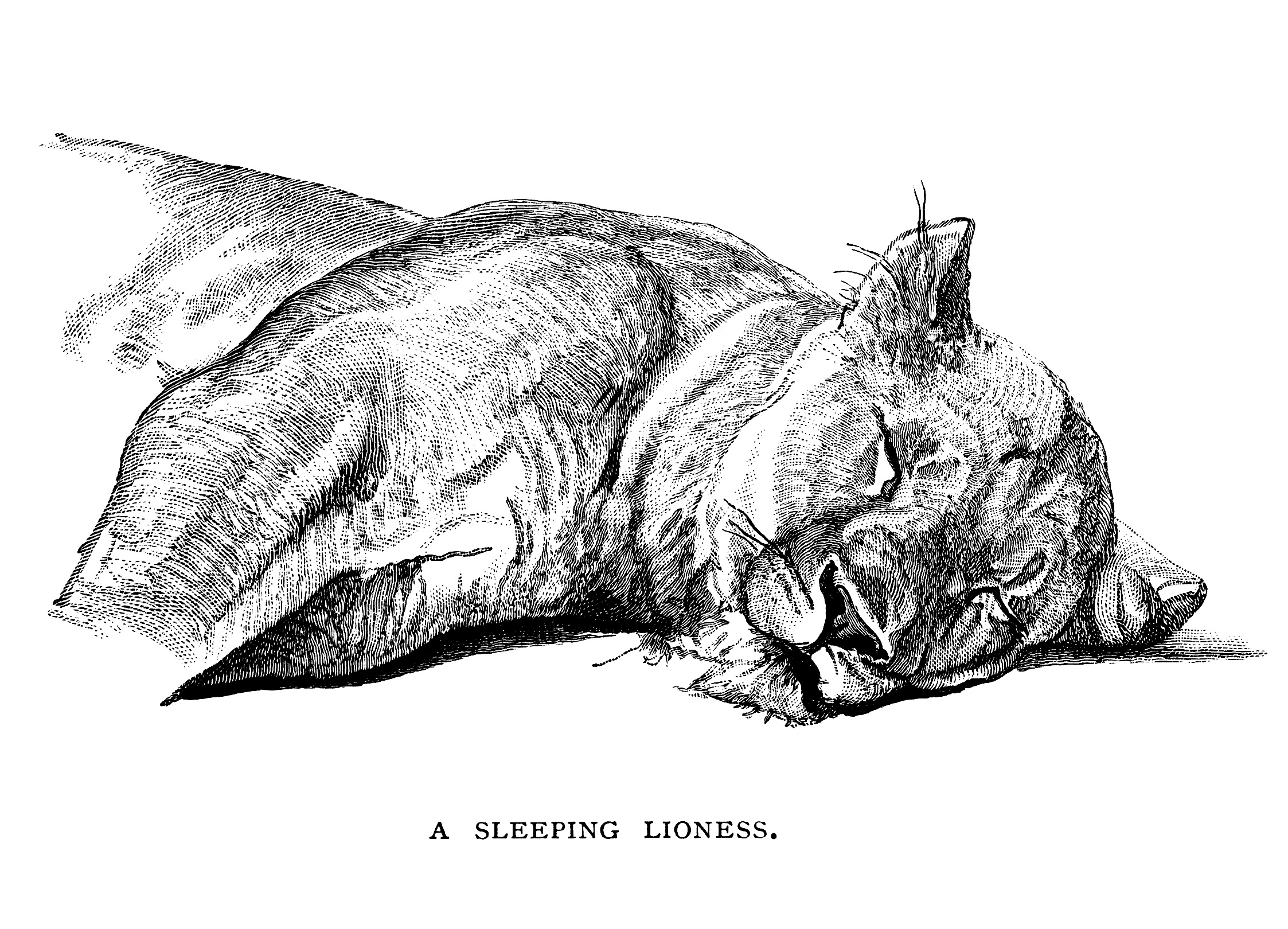In this detailed pencil drawing, we see a muscular lioness in peaceful slumber, identified by the text "A SLEEPING LIONESS" at the bottom center. The lioness is depicted lying on her side with her head tilted to the left, exposing her serene facial expression with closed eyes. Her two front legs are stretched out in front, showcasing her well-developed physique. Distinctive tufts of hair emerge from the inside of her visible ear, while the other ear lies against the ground. Whiskers protrude from her snout, and additional hair adorns her chin. The drawing is rendered in shades of gray with subtle white highlights, including a noticeable white patch beneath her ear extending to under her snout. This close-up illustration captures the essence of the lioness's tranquility and strength.